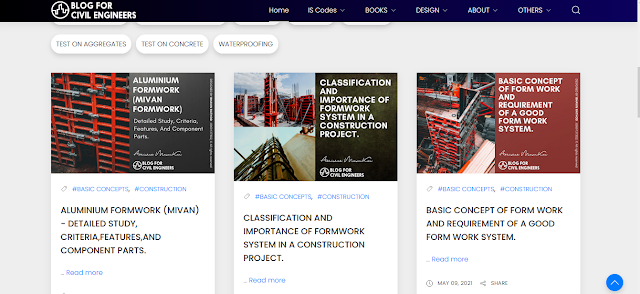The image is a screenshot of the "Blog for Civil Engineers" website. The logo consists of a simple skyline outline within a circle, followed by the text "Blog for Civil Engineers" with "Blog for" on the top line and "Civil Engineers" on the bottom line. 

The header starts out black on the left and gradually fades to almost purple on the right. At the top of the header is a menu with the options: Home, IS Codes, Books, Design, About, and Others, all of which have drop-down menus except for Home. There is also a magnifying glass icon for search functionality to the far right of the menu.

The webpage has been scrolled slightly downward, concealing five menu options in capsules but revealing the second line, which lists topics such as "Test on Aggregates," "Test on Concrete," and "Waterproofing."

Below this, there are three floating tabs. Each tab features an image on the left and a colored field with a capitalized header on the right. The first tab shows orange-painted I-beams at a construction site with the header "Aluminum Framework, Mavani Formwork." The second tab features two shots of a construction site with the header "Classification and Importance of Formwork Systems in a Construction Project," again showing predominantly orange colors. The third tab, also with an orange theme, has the header "Basic Concept of Formwork and Requirement of a Good Formwork System."

Beneath each of the images is text that reiterates the content: "Aluminum Formwork, MiVan Detailed Study, Criteria, Features, and Component Parts," along with similar descriptions for the other two tabs. There are also "Read More" options and dates at the bottom of the text.